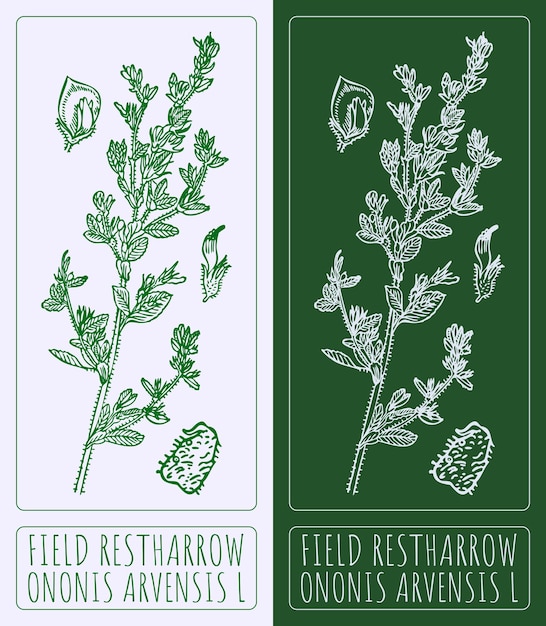This image features two vertically oriented color illustrations, each shaped like a bookmark and positioned side by side. A seam runs between the two bookmarks. The left bookmark has a white background with green text, while the right bookmark has a green background with white text. At the top of each bookmark, there is a detailed illustration of a leafy branch, surrounded by additional leaves and objects in an intricate etching or engraving style.

In a rectangular section with curved edges located at the bottom of each bookmark, the text reads: "field, rest arrow." Additionally, both the top and bottom portions of the bookmarks are adorned with the text "ONONIS ARVENSIS L.," which likely refers to the genus or Latin name of the plant depicted in the illustration.